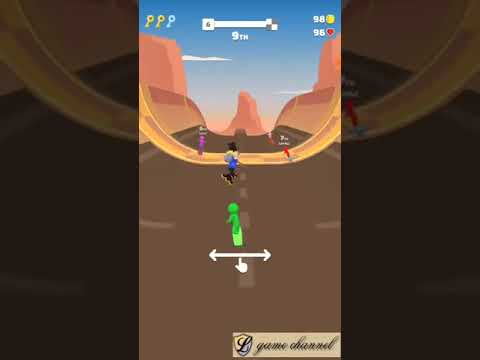The image captures a chaotic and vibrant scene from what appears to be a racing video game. The main focus is the central panel where a brown, streaked road stretches away from the viewer, bordered by reddish-orange walls on either side. A small green character, flanked by a white circle with a golden sword emblem and another gold circle, is moving down this road. Above the central panel, a progress bar, partially filled with yellow, indicates the player's position as fifth. In the top-left corner, three key icons, one golden and two white, are visible, while to the right, a series of numbers—321 in a yellow circle and 72 in a red circle—provide additional game data. An intriguing scene unfolds with a person seemingly hanging off-screen on the upper left. Both the left and right sides of the image are darkened, flanking the illuminated middle section. The entire setting is embedded in a brown canyon under a blue sky, enhancing the immersive quality of the game. The bottom right corner features a watermark in cursive, "Python L Game Channel," adding a touch of branding to the screen.